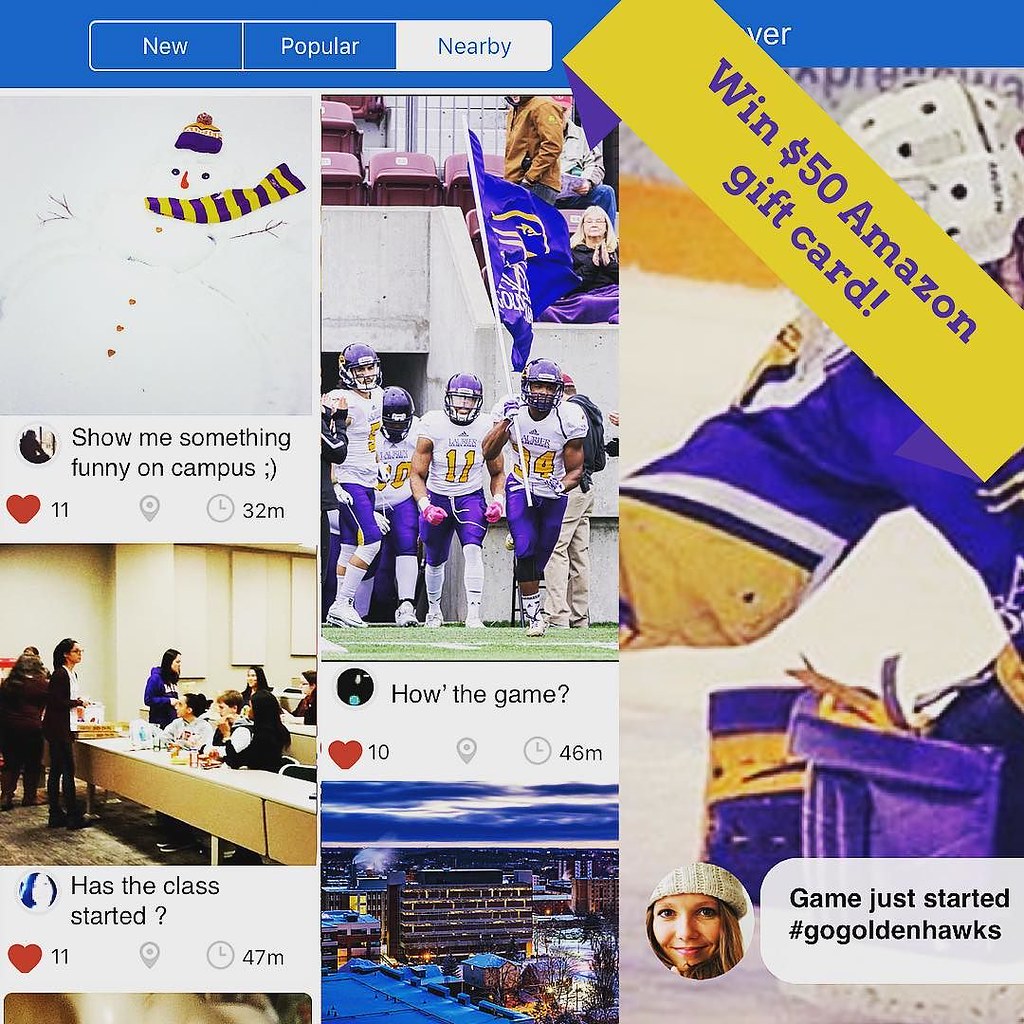This image is a dynamic, visually rich collage resembling a social media feed, likely an advertisement, showcasing various posts from platforms like Facebook or Instagram. The interface features a blue top border with three tabs: "New," "Popular," and "Nearby," with "Nearby" being highlighted. Dominating the top right corner, a diagonal yellow banner announces a chance to win a "$50 Amazon Gift Card."

The collage is divided into three columns of posts. The top left post shows a whimsical snowman, adorned with a blue and yellow scarf and hat, with the caption, "Show me something funny on campus," and it has received 11 hearts. Below it, a classroom scene prompts the question, "Has the class started?" It too has garnered 11 hearts and was posted 47 minutes ago.

The center column features a dynamic image of football players entering the field, led by a flag-bearer in white jerseys and purple helmets, captioned, "How's the game?" with 10 hearts. Beneath it is a dusky photo of a downtown area or campus building illuminated against a darkening sky.

The right column contains a striking photo of a hockey player in a blue jersey with yellow accents. Inserted into this image is a smaller picture of a girl in a woolen cap with the caption, "Game just started. #GoGoldenHawks," hinting at school spirit for a team named the Golden Hawks.

Overall, the collage integrates elements of representational realism with a vibrant social media aesthetic, creatively advertising campus life and events nearby.